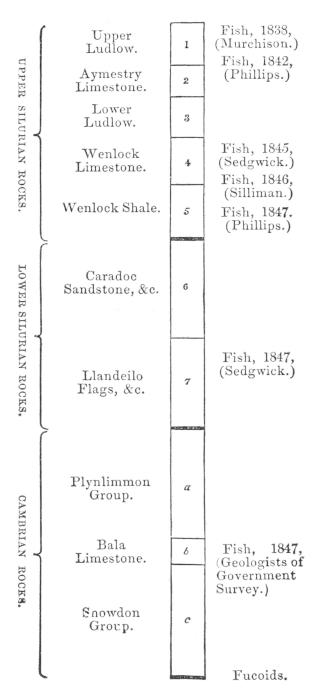The image depicts an old scanned chart from a geology textbook, detailing different rock categories and their corresponding time periods. It showcases a vertical scale from 1 to 7, followed by the letters A, B, and C. The chart categorizes rocks into three distinct periods: Upper Silurian Rocks, Lower Silurian Rocks, and Cambrian Rocks. Within the Upper Silurian period, the subcategories are Upper Ludlow, Aymestry Limestone, Lower Ludlow, Wenlock Limestone, and Wenlock Shale. The Lower Silurian period includes Caradoc Sandstone and the Llandeilo Flags. The Cambrian period is divided into the Plinlimon Group, Bala Limestone, and Snowdon Group. The chart also contains annotations implying the presence of fish within these rock layers, and the timespan covered is from 1838 to 1874.